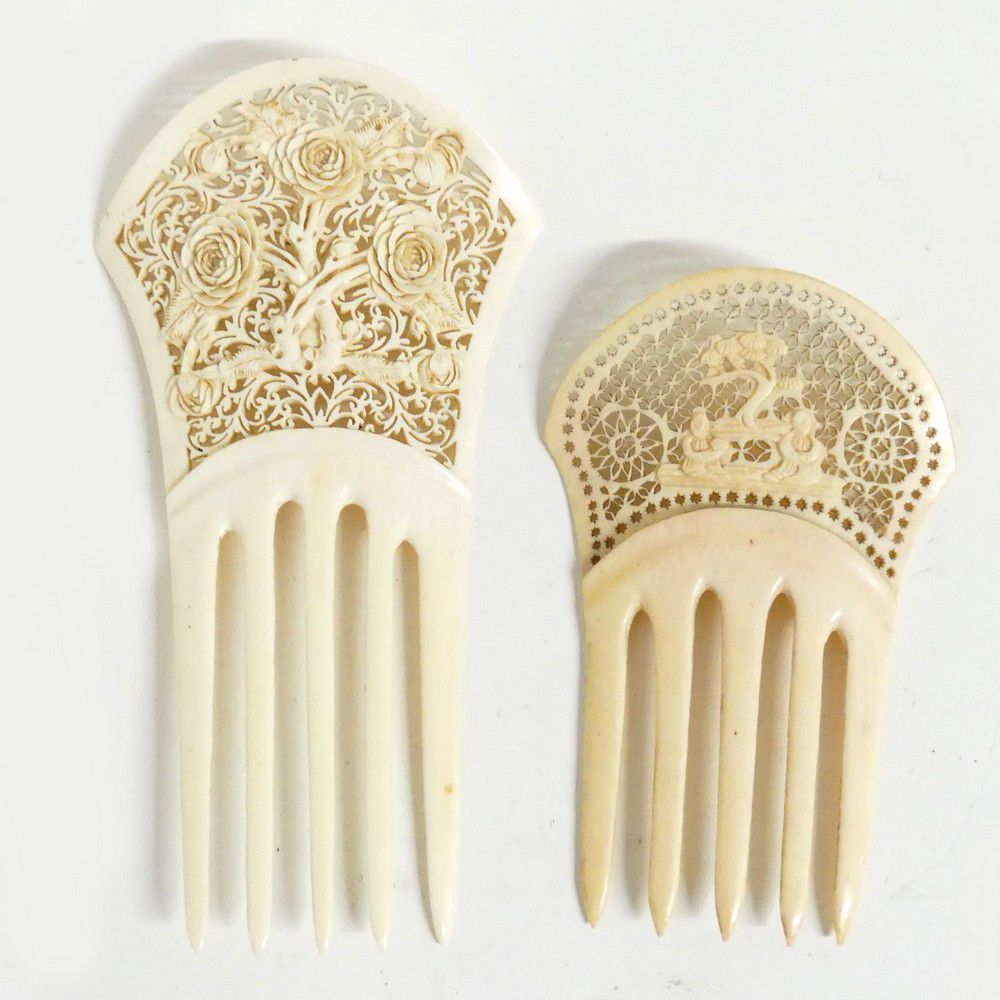The picture features two intricately carved, antique hair combs laying side by side on a white surface. Both combs are white, though they exhibit different shades; the left comb is a lighter cream while the right one has a slightly darker, beige hue. Each comb has five prongs at the base. The left comb is taller and showcases an elaborate top with three carved roses, emphasizing its floral motif. The right comb, shorter in stature, displays a detailed carving of a bonsai tree with two small characters sitting underneath. The material of the combs appears to be either plastic or bone, possibly ivory, adding to their vintage charm as fashion accessories.